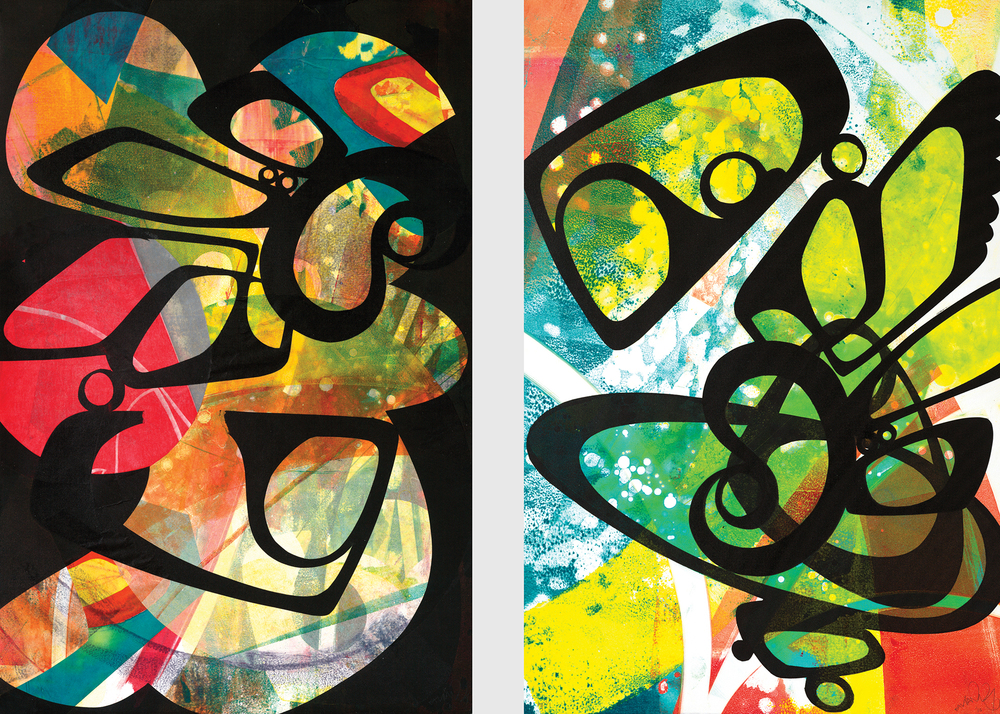The image features two side-by-side abstract paintings, both vertical rectangles, separated by a thick vertical light gray bar. The painting on the left has a predominantly black background with swirling black patterns and vibrant, fan-like shapes interspersing through it. The colors in these shapes include bright hues of orange, blue, red, yellow, green, and white, creating a dark yet colorful composition accented by black lines. In contrast, the painting on the right is far brighter, featuring a lighter, more colorful background with splashes of white, blue, red, yellow, and green. Black lines weave thickly through this painting as well, but here they serve to accentuate the colorful backdrop rather than dominate it. Together, these paintings form a striking pair of complementary opposites: one dark with bursts of color and swirling black lines, and the other vividly colorful with prominent black swirls and lines intermingling with the brightness.